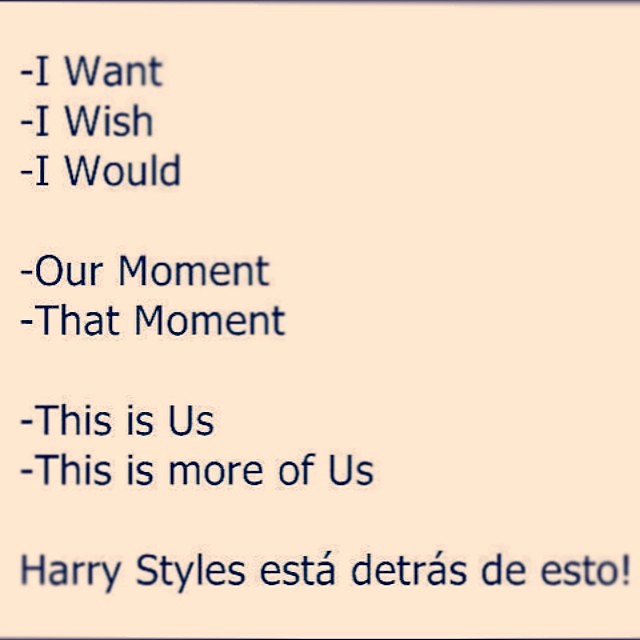The image features a minimalist, beige background with printed black text in a list format. The statements, separated by dashes, read: "I want," "I wish," and "I would." This is followed by a few spaces, then "our moment," "that moment," "this is us," and "this is more of us" spaced similarly. At the bottom of the image, in bold navy blue text, it reads, "Harry Styles está detrás de esto," with an acute accent over the 'á.' There are no people or additional elements in the image, emphasizing its plain and informational design.